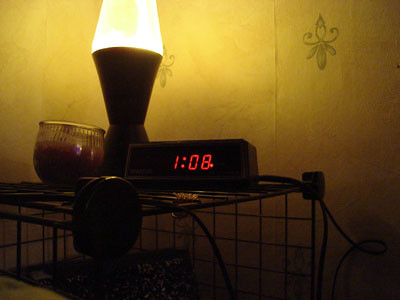This close-up image features a vintage-style, rectangular alarm clock with a digital display reading "1:08" in red. A small dot at the bottom right of the '8' indicates that the alarm is set. The clock rests atop a black wire dog cage. To its left, a small round jar containing a candle adds a touch of coziness. In the background, a white-lit lava lamp provides ambient lighting, casting a soft glow on the scene. The wallpaper behind the setup has a tan color with a subtle, small floral print, adding a classic and textured element to the overall composition.